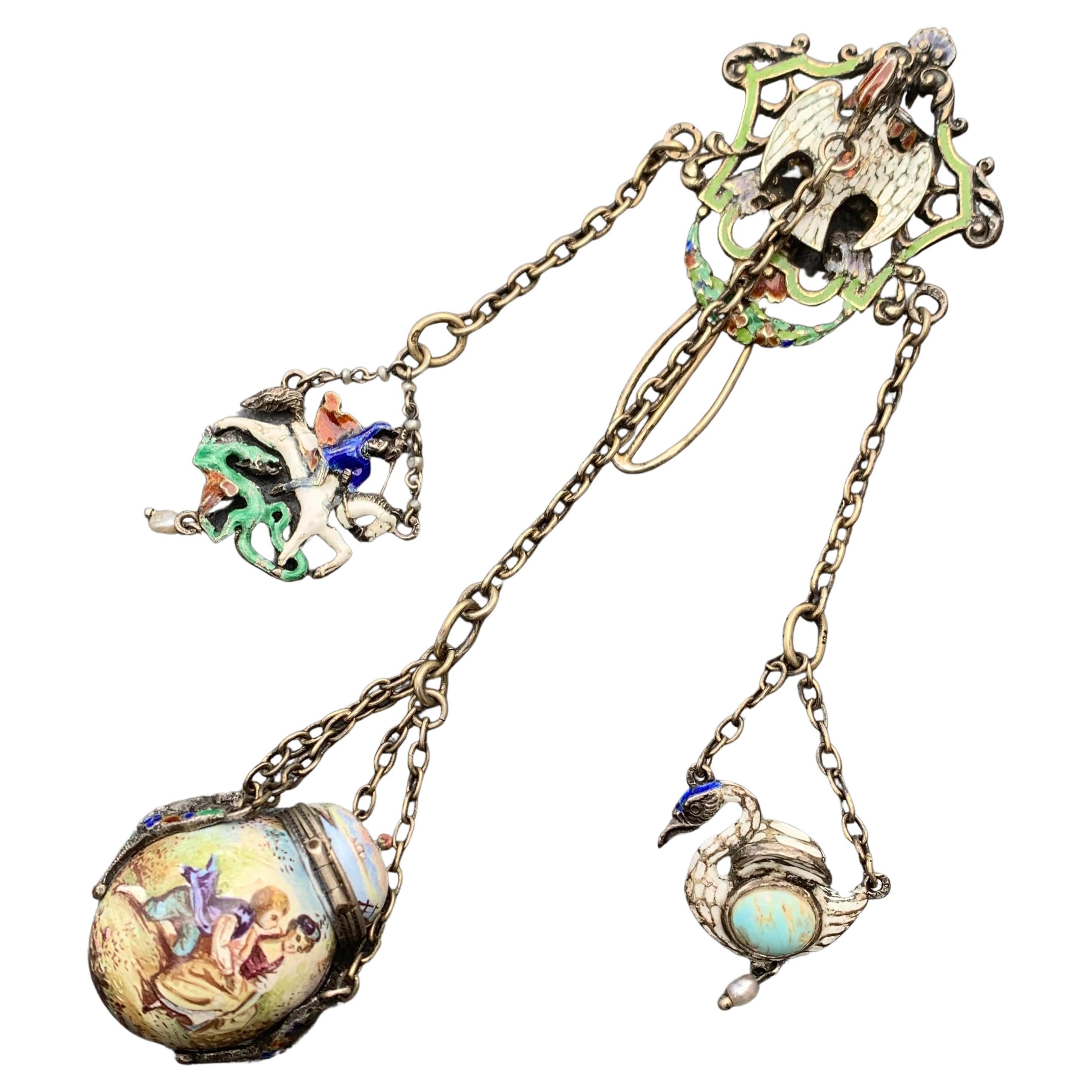This intricately detailed necklace features an ornate central pendant resembling a skull with a crown, flanked by two shorter gold chains and a longer one in the middle. The central pendant’s peculiar design has a bird-like figure etched into its golden surface, adding an air of mystique. The pendant culminates in a delicate silver piece that transitions into a thin ring, anchoring the first of the three cascading chains.

Suspended from the left chain is a pendant with a charming depiction of a woman, adorned in vibrant colors of green, beige, pink, and blue, adding a touch of whimsy and fantasy to the piece. The right chain supports an elegant pendant of a crane, showcasing detailed artistry with a blue head, white neck, and tail. This bird charm is embellished with a striking blue stone set in the center, adding to its allure.

The middle chain, the longest of the three, culminates in what appears to be a pendant or locket featuring a detailed depiction of a woman and child, primarily colored in hues of yellow and blue. All three chains and their respective pendants are connected to the main body of the necklace with stabilizing rings, adding to the piece's structural integrity and visual balance. The combination of these elements renders the necklace not only a piece of jewelry but a miniature work of art.